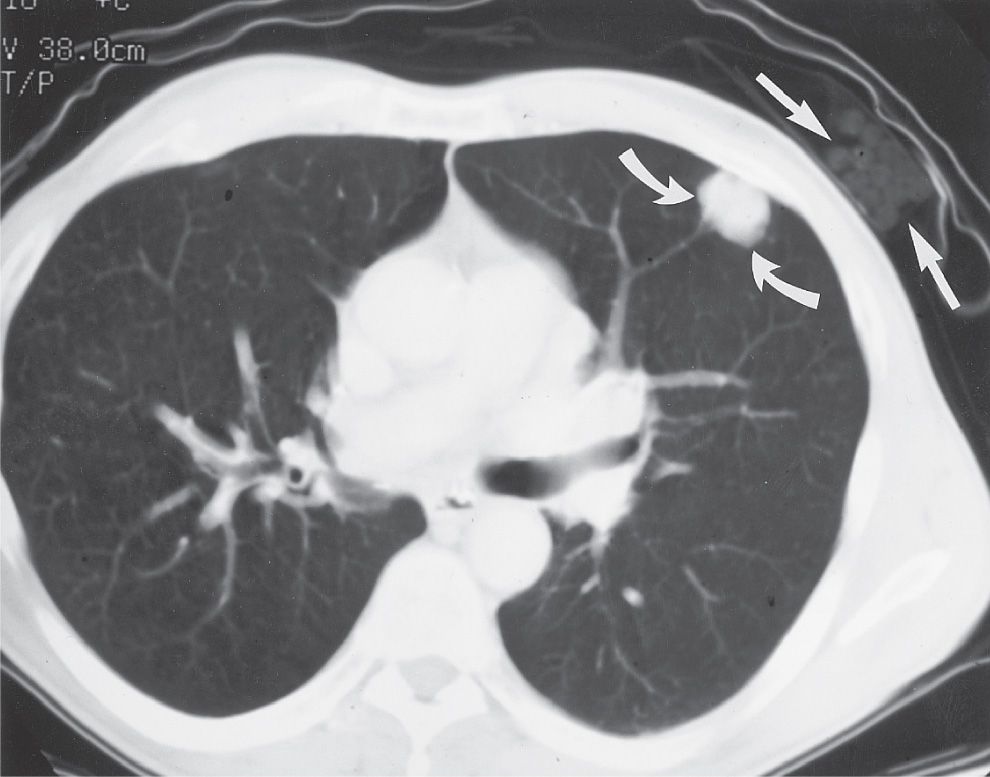This black and white CT scan, oriented in landscape, features a detailed view of the lungs highlighting a pneumothorax condition. The central region of the lungs shows white areas surrounded by kidney-shaped dark sections on either side. A white membrane outlines these kidney-shaped lung sections, with an additional gray and black membrane layer encircling the entire structure. Within the central white membrane area, there are two white arrows, one pointing upwards and the other downwards, and outside this white border, another light gray mass can be seen with additional arrows pointing towards it. Technical information, partially cut off, appears in the top left corner of the image, displaying measurements such as 38 centimeters. Lastly, a round white mass is visible at the top right, highlighted by two arrows pointing towards it, emphasizing the anatomical and technical details depicted in this CT scan.